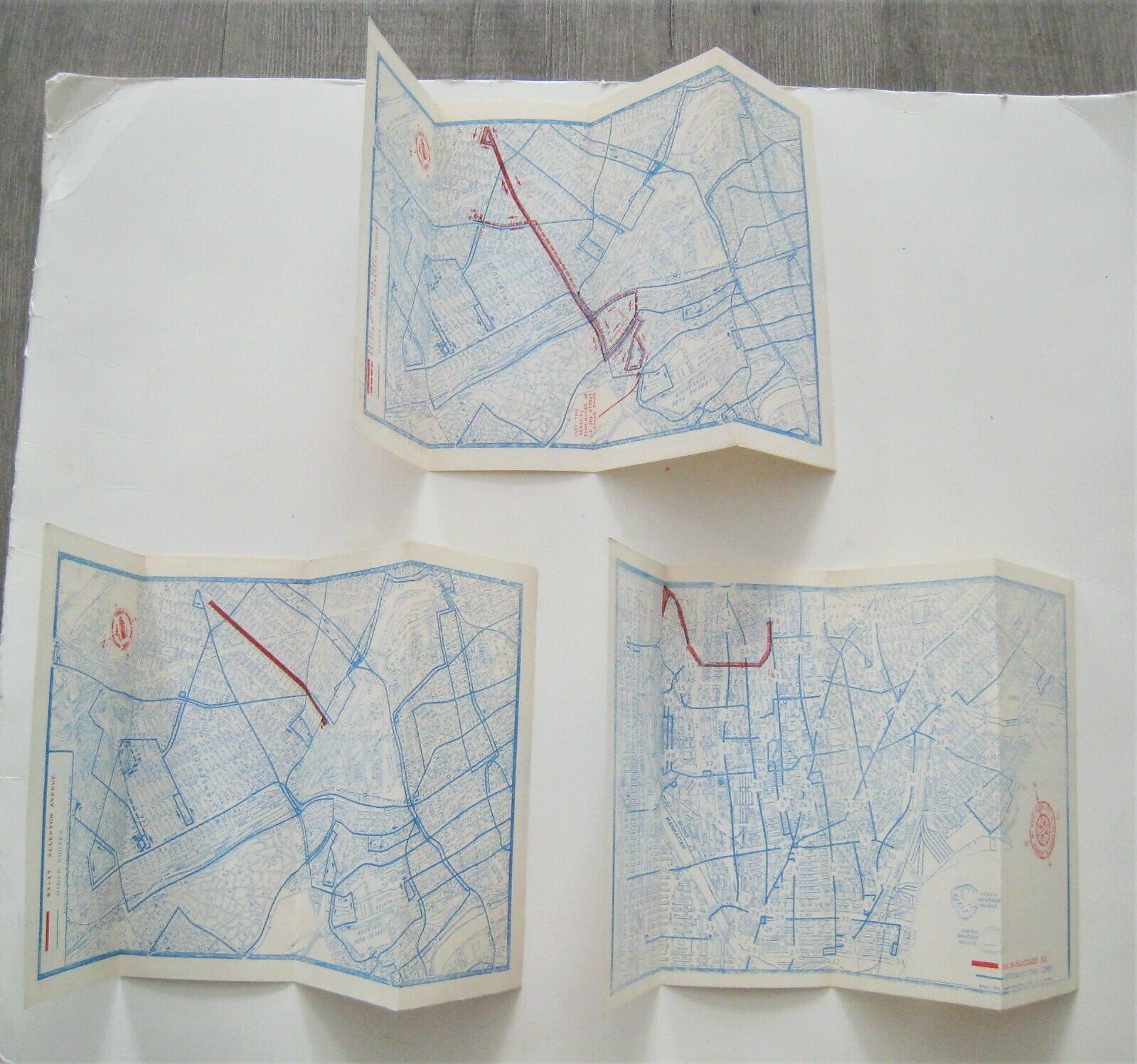This image is a color photograph taken indoors, showcasing a wooden table with a grayish tint, possibly a gray fake wood. The grains of the wood are visible in the background, providing a textured surface for the items on top. Lying on the table is a large white piece of cardboard-like paper, which is somewhat curled at the edges, casting shadows due to overhead lighting.

Spread across the white paper are three small, completely unfolded maps. These maps appear to depict an inner-city setting, illustrated with a network of blue lines suggesting streets or routes, and certain areas shaded in blue. Each map features a prominent red line, which varies in length and pattern across the maps, potentially indicating specific pathways or destinations. Additionally, all three maps include compass stamps denoting north, south, east, and west directions.

The overall scene gives the impression of a methodical layout, possibly for navigation or planning purposes, and while the exact nature of the maps isn't clear, they resemble street maps with intricate designs meant for travelers or city planners.